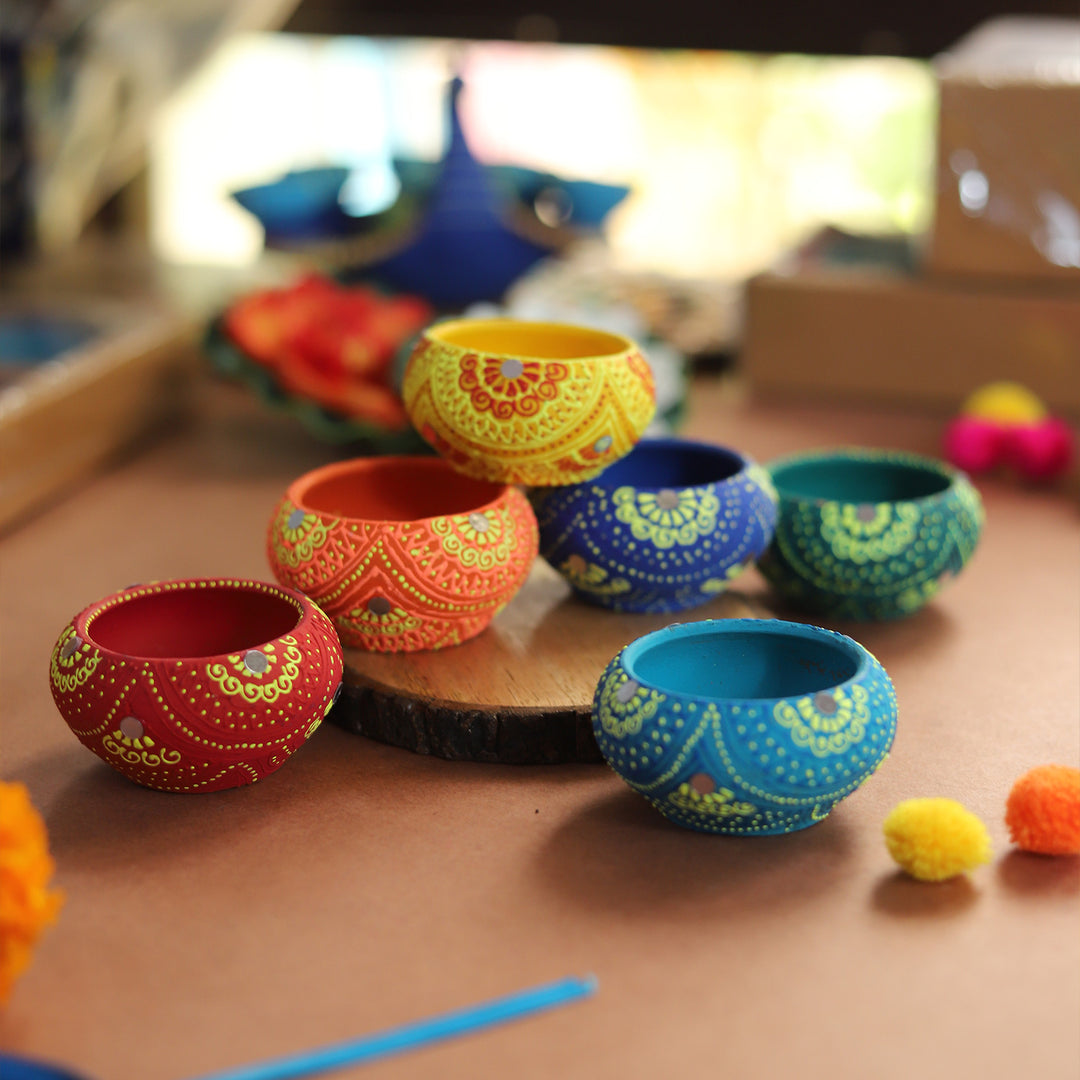The image depicts a craft setup on a medium brown table or desk, featuring an assortment of tiny, ornate ceramic bowls adorned with colorful floral and geometric patterns. Central to the square picture is a glossy circular wooden tray with bark edging, on which three ceramic bowls are neatly stacked: an orange bowl at the base, topped by a blue one, and capped with a yellow bowl featuring red or orange flowers. Surrounding the tray are three more bowls in vibrant hues—red with yellow flowers, blue with yellow flowers, and a light blue—with each featuring intricate dot and pattern designs. Scattered on the table are bright orange and yellow cotton balls adding additional splashes of color. The background is slightly blurry, revealing more art supplies and additional bowls, with a glimpse of a window at the top contributing natural light to the artistic scene. At the bottom edge of the image, the tip of a blue paintbrush handle is partially visible, hinting at ongoing creative activities.